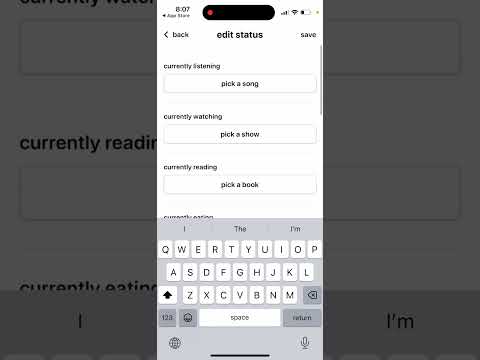This image appears to be a screenshot showcasing a smartphone interface on a larger, darkened desktop background, highlighting how the webpage would appear on a mobile device. In the center, prominently featured is the smartphone screenshot. 

At the top left of the image, the time reads "8:07," and at the top right, a battery icon indicates the charge level is approximately one-fourth full. Centered at the top of the screenshot is a black, sideways oval with a red dot on the left, potentially obscuring the website's name or a notification indicator. 

Directly beneath this, there's a navigation bar with an "Edit Status" label, flanked by a back button on the left and a save button on the right. Below this bar, the interface displays sections for the user's current activities: 

- "Currently Listening" with an option to "Pick a song."
- "Currently Watching" with an option to "Pick a show."
- "Currently Reading" with an option to "Pick a book."

This interface seems designed to let users update and share their current media consumption status, acting as a profile page to display what they're currently engaged with in terms of listening, watching, or reading.